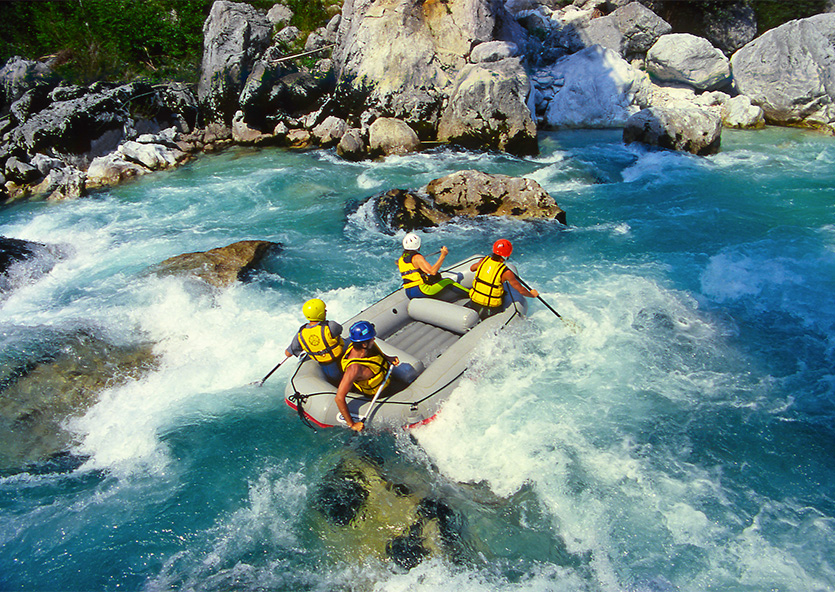An aerial photograph captures an exhilarating whitewater rafting adventure as four rafters navigate the crystal-clear turquoise river. The rafters, positioned two in the front and two in the back within a nine-foot light gray raft, are clad in yellow life jackets with helmets in white, red, yellow, and blue. Each rafter grips an oar, working to steer the raft around protruding gray rocks and through the churning white waves. The scene is dynamic, with the raft turning to the right to avoid a rocky outcropping. The left-hand side of the image shows the rocky shore and a backdrop of trees in the top left corner, while the right side is dominated by the turbulent water rapids. This vivid image captures a moment of teamwork and adventure amid nature’s raw beauty.